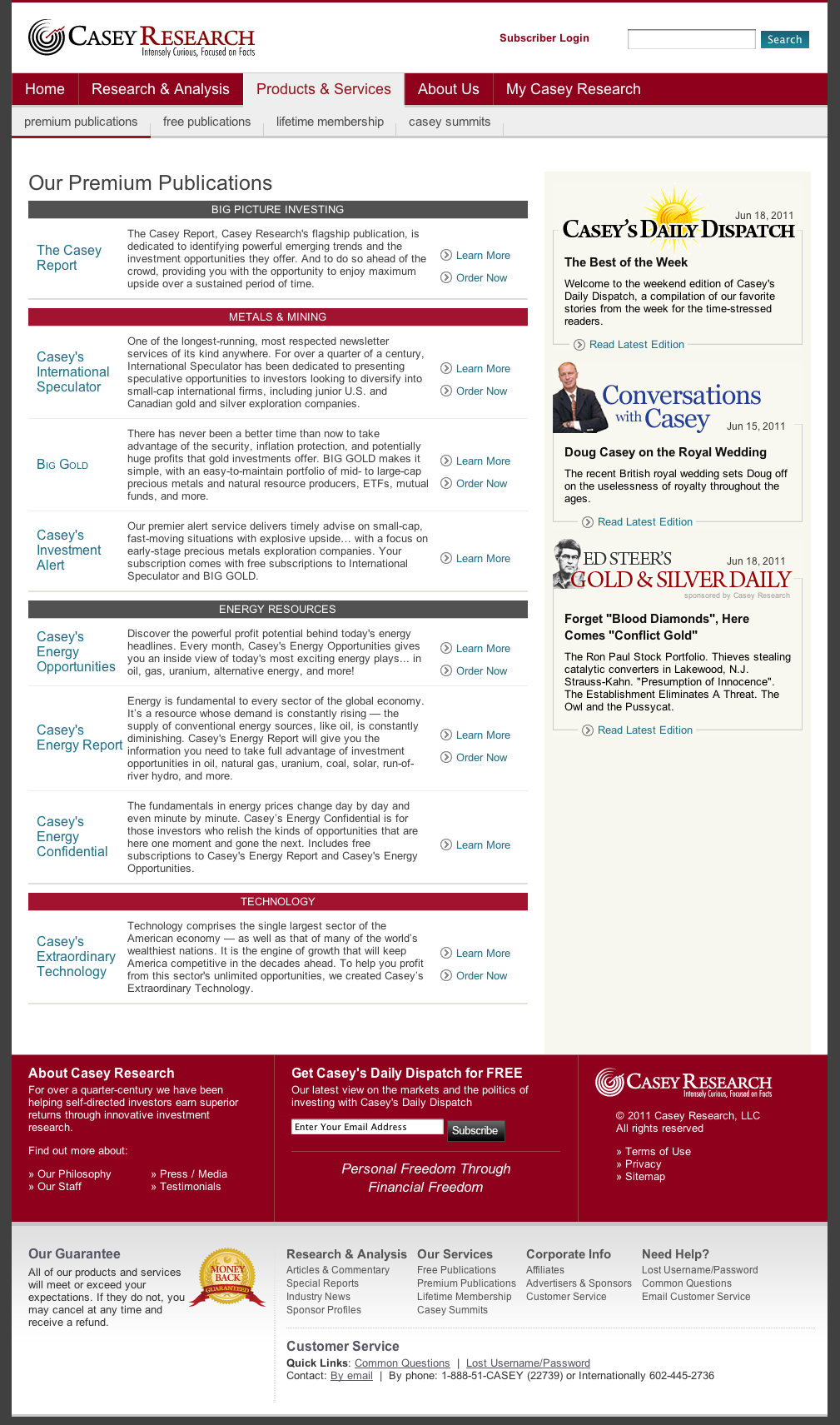KC Research: Where Curiosity Meets Insight

This detailed image showcases the website homepage of KC Research, a company renowned for its dedication to delivering in-depth research and analysis across various sectors. The prominently displayed slogan, "Intensely Curious, Focused on Facts," encapsulates KC Research's commitment to thorough and factual investigation. 

The homepage is neatly categorized into sections such as "Home," "Research and Analysis," "Products and Services," and "About Us." It provides various user access points including "My KC Research," "Subscriber Login," and "Lifetime Membership." 

For those interested in publications, the site offers both "Premium Publications" and "Free Publications." Among the premium offerings are "Big Picture Investing" and "The KC Reports," the latter being KC Research's flagship publication. This flagship report focuses on identifying powerful emerging trends and the lucrative investment opportunities they present, all while aiming to stay ahead of the crowd to maximize long-term gains.

The research scope spans multiple industries including Metals & Mining, Energy Resources, and Technology, signifying KC Research’s broad yet detailed expertise in these fields.

Additional features on the website include information on "KC Summits," providing a more interactive and engaged platform for subscribers and members. Overall, the homepage efficiently communicates the wealth of resources and insights available through KC Research, making it a valuable tool for informed investors and analysts.